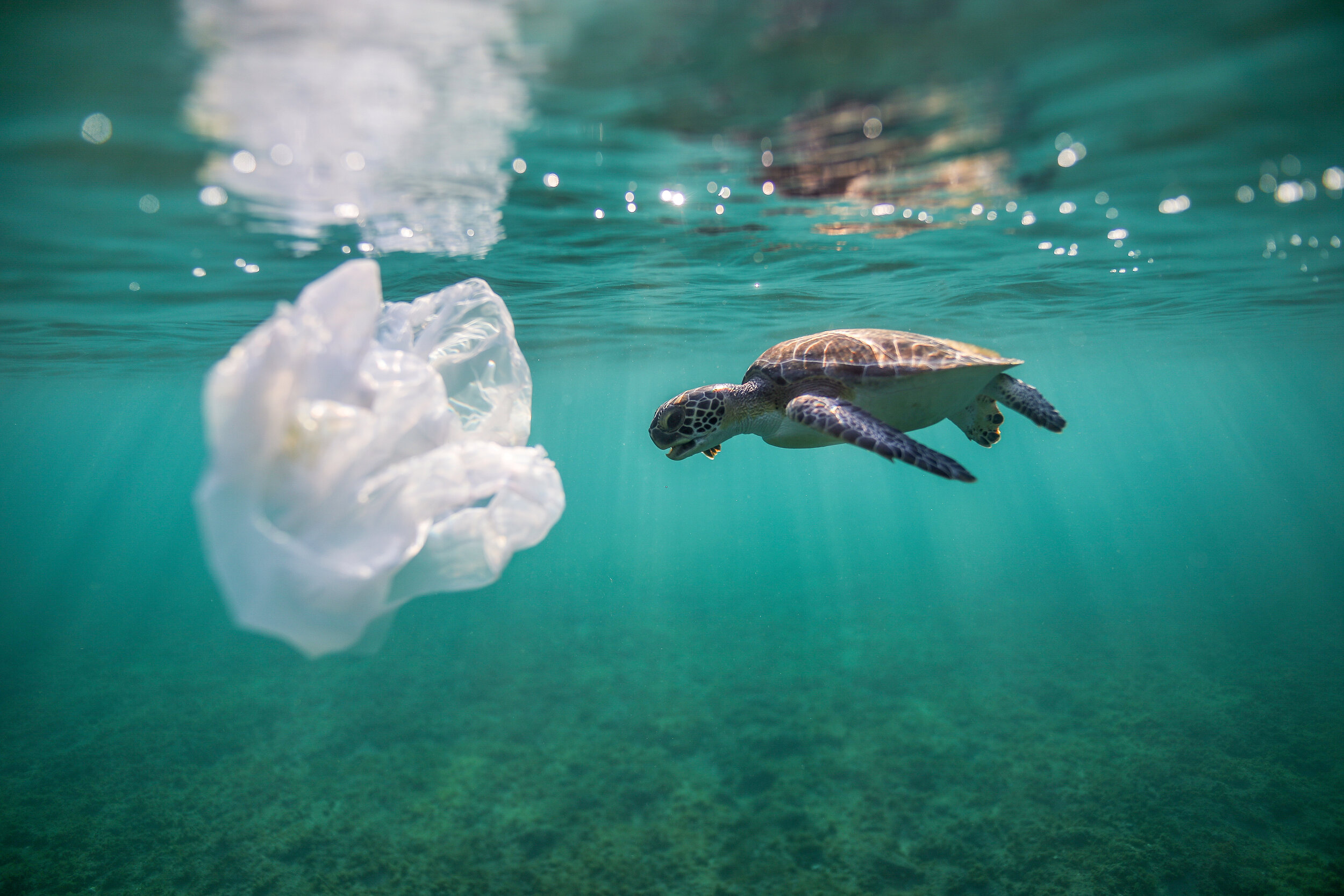In this detailed underwater photograph, we see a vivid depiction of a small sea turtle swimming near the surface. The image, rectangular in shape and approximately five by four inches, captures the turtle with its arms and legs fully extended as it glides through the greenish-blue, sea foam-colored water, tinted by sunlight rays penetrating from above. The turtle's brownish back and white underside, along with its open mouth and small square markings on its head, are clearly visible. In front of the turtle, a white plastic bag floats, possibly mistaken by the turtle for a jellyfish. Above them, the surface of the water breaks, offering a reflective quality where the turtle and the bag are mirrored, lined with tiny bubbles and light dots. The seafloor below, occupying the bottom third of the image, appears jagged and rocky, dotted with bits of coral and plant life, completing this mesmerizing underwater scene.